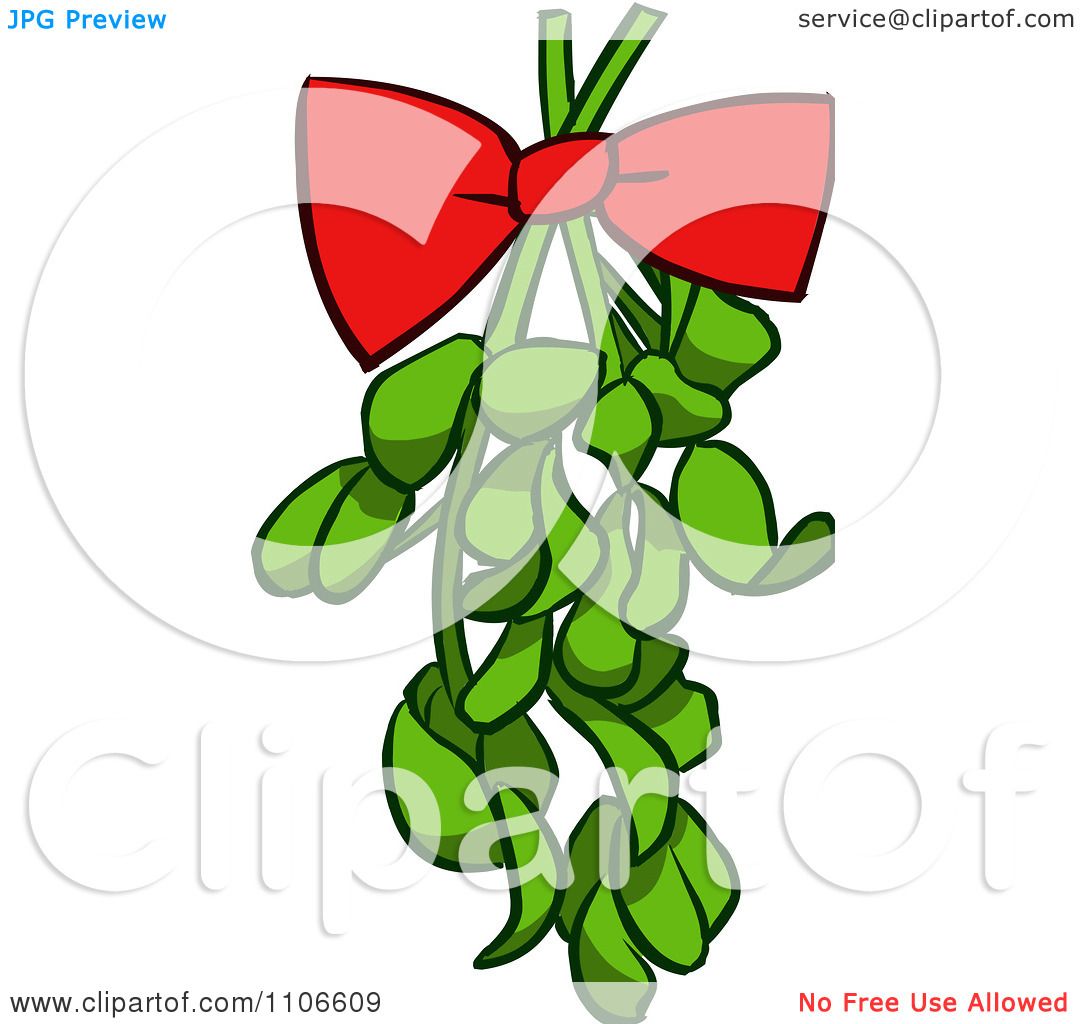This image is a digitized clip art drawing of mistletoe, characterized by its green leaves and a red bow tied in a knot at the center. The bow and leaves are framed with a black outline, enhancing the clarity of the digital artwork. The mistletoe appears to be crisscrossed by two tree branches, with the stems extending from the top to the bottom of the image, surrounded by green leaves. The image contains several watermarks: the clip art symbol (resembling an infinity sign) prominently displayed and slightly faded around the bow and leaves, and the text "clipartof" also faded in the background. Additional text overlays include "JPG Preview" at the top left, "service at clipartof.com" at the top right, "www.clipartof.com/1106609" at the bottom left, and "no free use allowed" in red at the bottom right, signifying its proprietary status. The setting suggests a Christmas theme, supported by the red and green colors commonly associated with the holiday season. The URL and additional text reiterate the availability and usage restrictions of the clip art from the website www.clipartof.com/1106609.